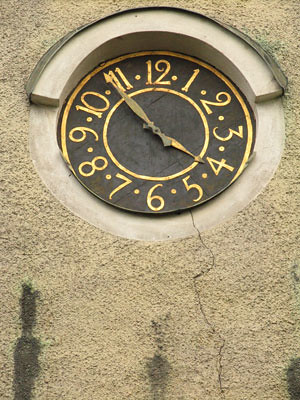This outdoor photograph features a clock face embedded into a rough-surfaced wall, likely made out of adobe or stone with a light tan color. The wall, covered in stucco with a few plants and patches of moss, shows signs of age with a prominent crack running vertically. The focal point of the image is the clock, ensconced in a circular concrete frame that adds dimension with stepped levels and a concrete ledge at the top. The clock face itself is a dark color, possibly black or dark brown, and features stylized gold numbers from 1 to 12. Two concentric golden circles add intricate details to the face. Both the minute and hour hands are gold, indicating a time of approximately 4:54 PM. The clock face shows some wear and a dent at the bottom, hinting at its long-standing presence in the wall.